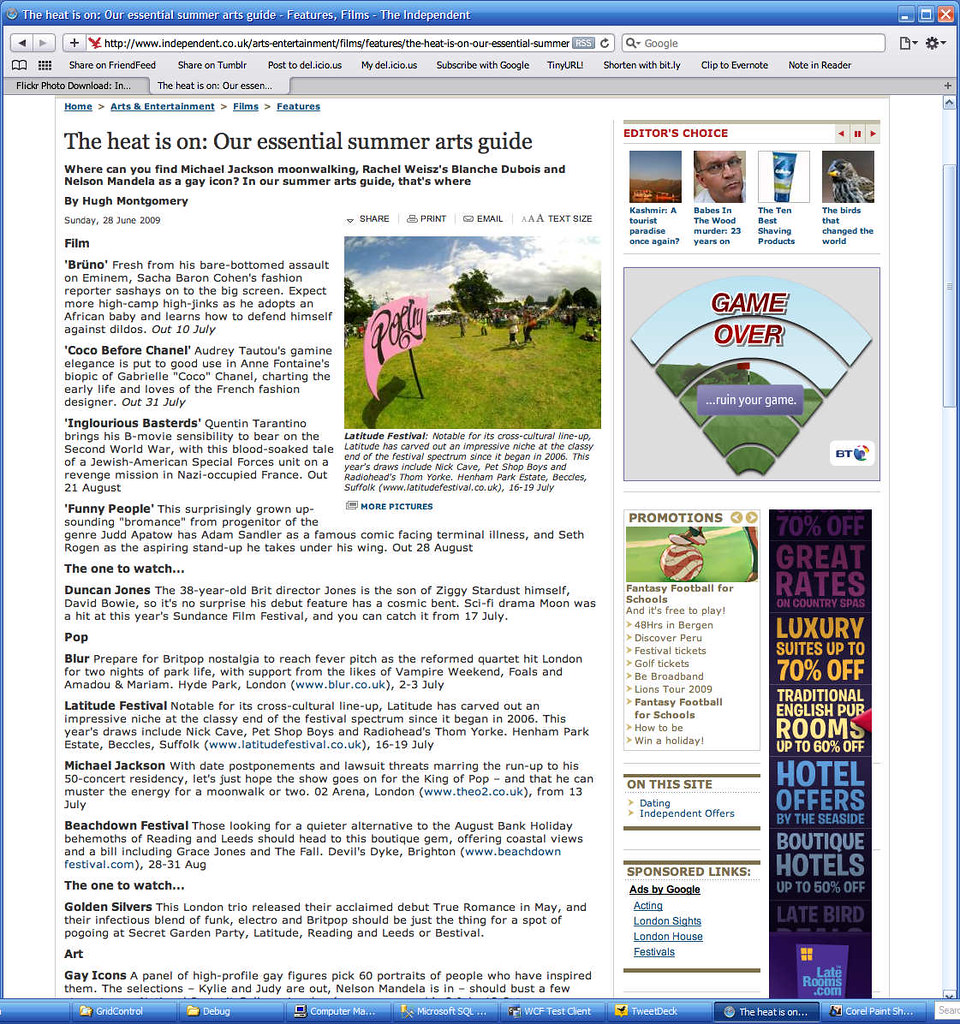**Desktop Screenshot of Essential Summer Arts Guide Article (June 28, 2009)**

The image captures a detailed screenshot of a desktop computer displaying an article titled *"The Heat Is On: Our Essential Summer Arts Guide"* authored by Hugh Montgomery. The article, dated Sunday, June 28, 2009, teases an exciting summer lineup, posing the intriguing question: "Where can you find Michael Jackson moonwalking, Rachel Weisz, Blanche DuBois, and Nelson Mandela as a gay icon? In our Summer Arts Guide, that's where."

### In the Film Section:
- **Bruno**: Sacha Baron Cohen's flamboyant fashion reporter, fresh from a notorious stunt involving Eminem, makes his big-screen debut. Expect high-camp antics as Bruno adopts an African baby and defends himself against dodos. Release date: July 10.
- **Coco Before Chanel**: Audrey Tautou stars in Anne Fontaine's biographical film, bringing to life the early years and romances of Gabrielle "Coco" Chanel. Release date: July 31.

### Additional Mention:
An image within the article highlights the Latitude Festival, featuring green grassy space and a sign reading "Poetry." Renowned for its eclectic and sophisticated mix since its inception in 2006, this year's festival promises exciting performances by Nick Cave, Pet Shop Boys, and Thom Yorke of Radiohead. Dates: July 16-19.